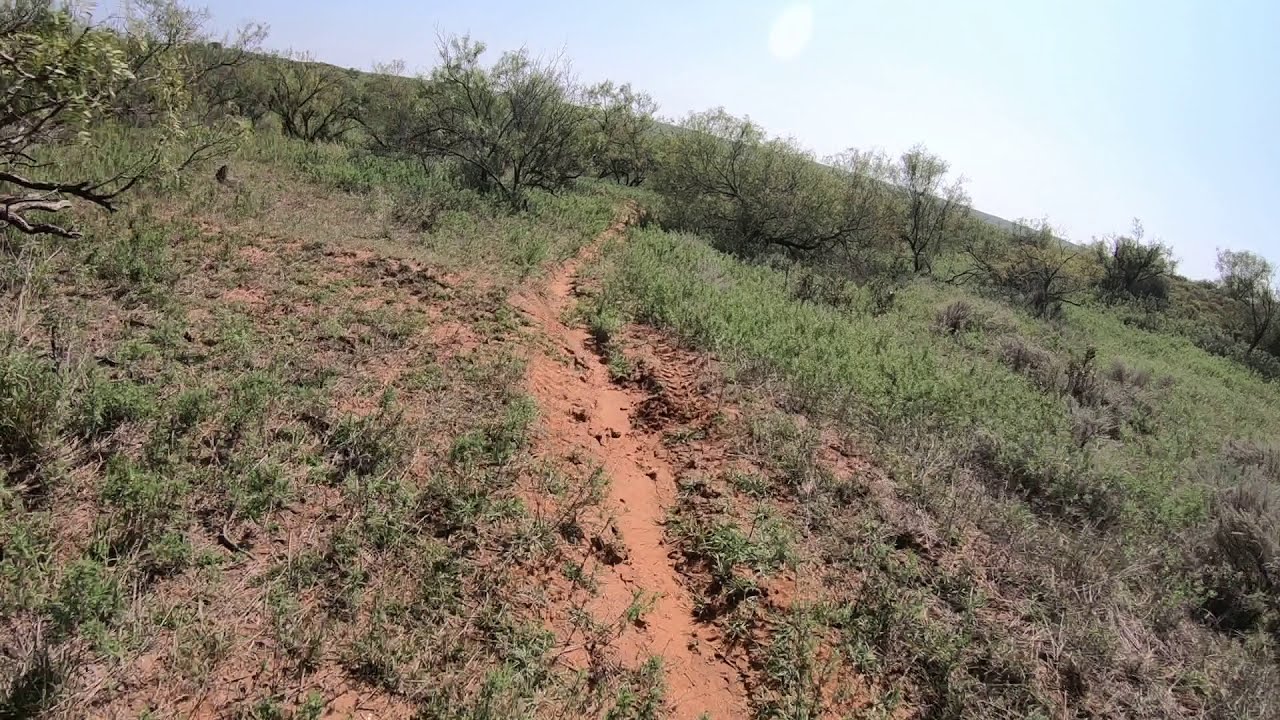The image depicts a remote and serene landscape, dominated by a narrow, reddish-brown dirt path that meanders through a field of varied green vegetation and patches of dry brush. Sparse trees and bushes are scattered throughout the scene, lending to its natural and unspoiled appearance. The trail, muddy in places, gently slopes upward toward a small hill in the distance, which takes up a significant portion of the background. The sky above is a clear, light blue, and the bright sunlight bathes the entire landscape, highlighting the different shades of green and brown in the grass and plants. The area appears devoid of human presence, emphasizing its tranquility and untouched beauty.